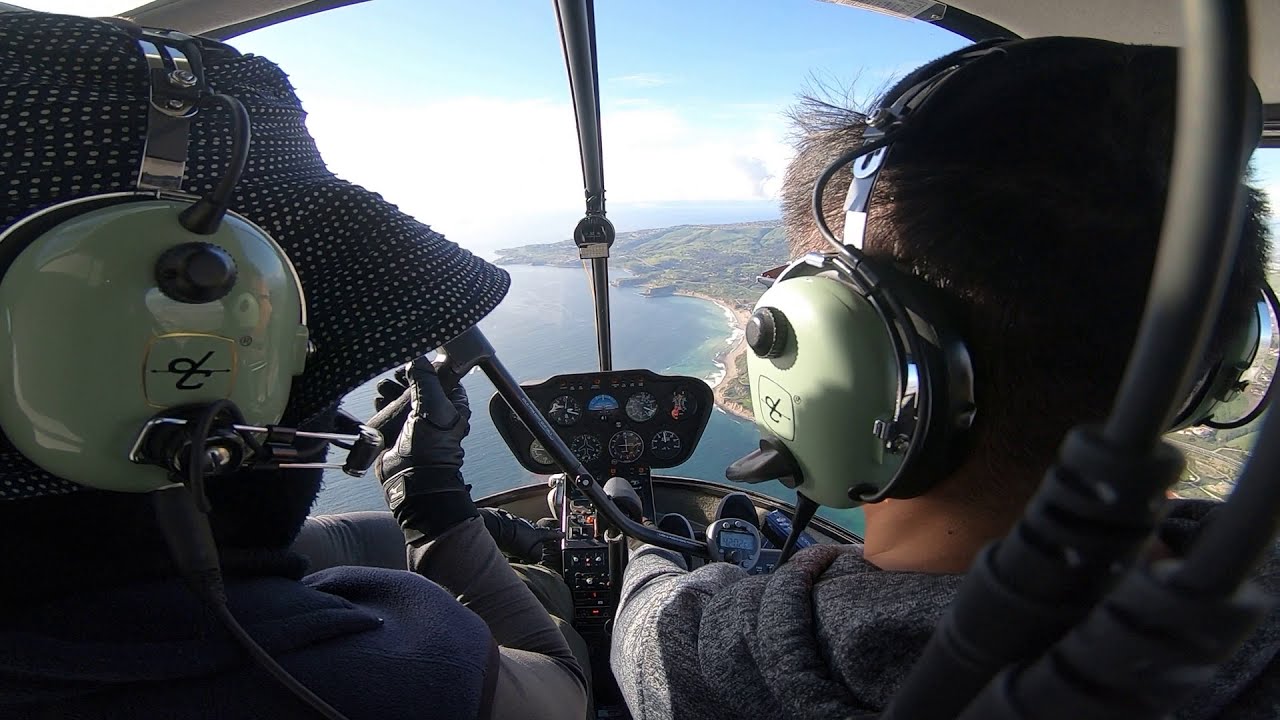This horizontally aligned rectangular image captures the interior of what appears to be a helicopter cockpit, seen from behind the pilot and co-pilot. Both individuals wear silver-cupped headsets with black wiring and headbands. The pilot on the left sports a black bucket hat with tiny white polka dots and is dressed in a blue vest over a long-sleeve gray shirt. He also wears a black glove on one hand while holding a black tool attached by a cord to the dashboard. The co-pilot on the right, with short spiky black hair, is clad in a gray hoodie and appears to touch the dashboard as well. The cockpit is filled with various dials, odometers, and controls necessary for flight. Through the windows, a picturesque scene unfolds: a vivid blue sky speckled with a few white clouds mirrors off the water below, with glimpses of land, a narrow beach line, and possibly some distant buildings and bushes, stretching across the horizon.